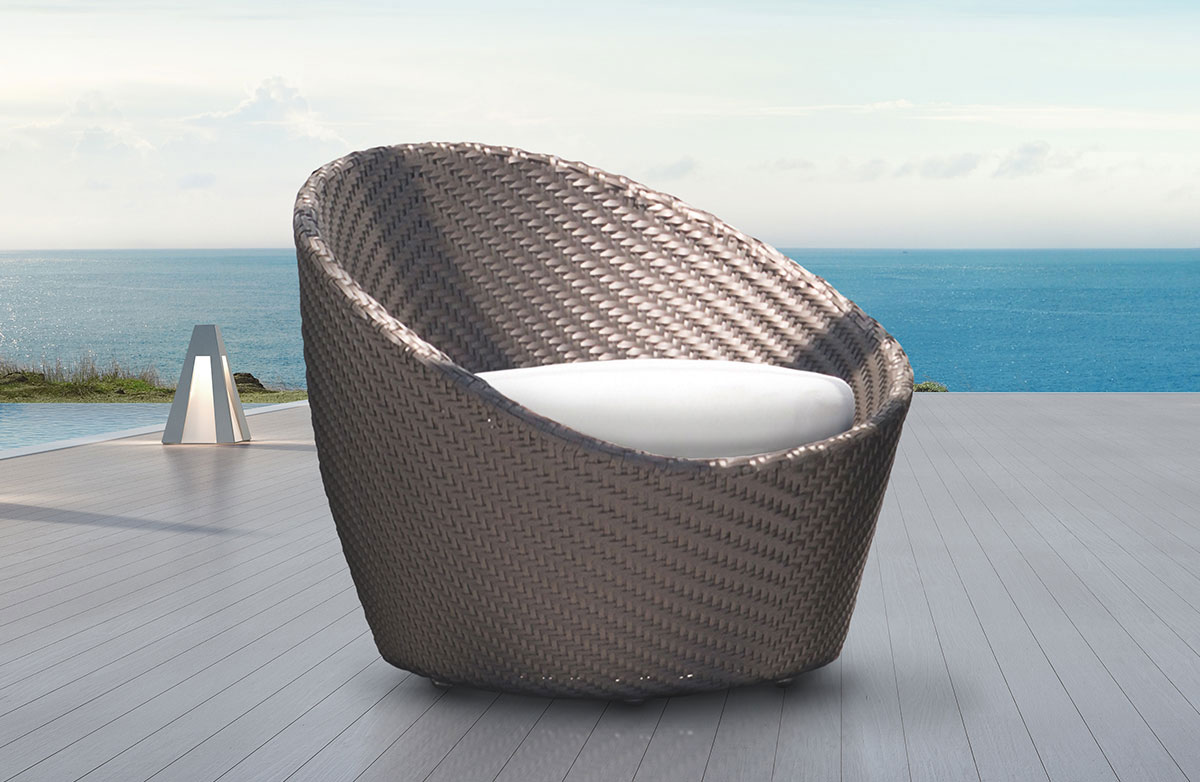The image depicts a silver, round-topped wicker chair with a white cushion, positioned outside on a gray wooden deck. To the left of the chair on the deck is a triangular light fixture sitting on the ground. The backdrop features a patch of green grass leading to the expansive view of a large body of water, which transitions from a striking blue on the right to grayish hues on the left. Above, a partly cloudy sky spreads across the horizon, casting a bright yet diffused light over the scene. The overall ambiance suggests a serene outdoor setting, reminiscent of a boardwalk near the sea, with the chair invitingly placed to take in the view.